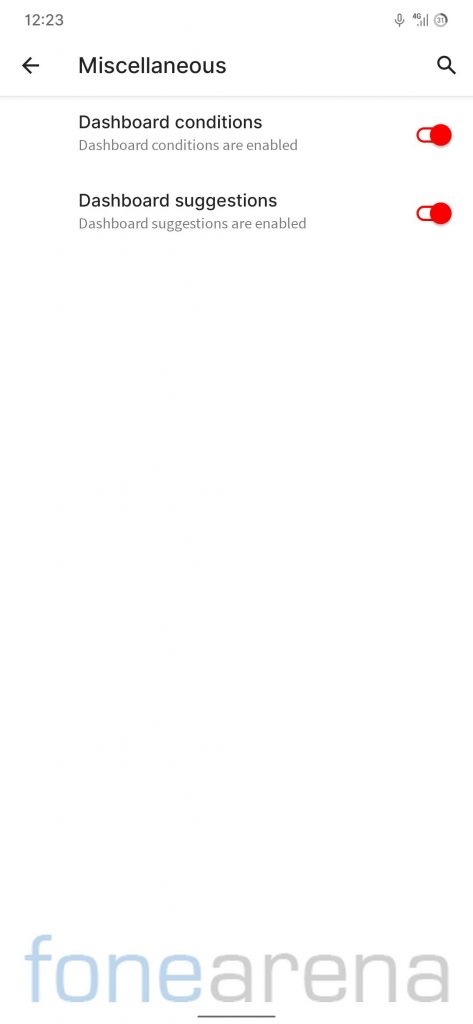The image displays a dashboard interface featuring various settings and options. Prominently, there are two toggles labeled "Dashboard Conditions" and "Dashboard Suggestions," both of which are enabled, indicated by red buttons slid to the right. The current time, "12:23," is displayed at the top of the screen. Above this, there is an icon resembling a microphone, suggesting a voice input feature. Adjacent to it, a magnifying glass icon denotes a search function. At the bottom center of the dashboard, the text "phone arena" is visible, with "fone" in blue and "arena" in a greyish-blue color; "a" and "r" in "arena" are underlined, all formatted as one single word. Additional symbols are present at the top of the screen, though their specific functions are not immediately clear.